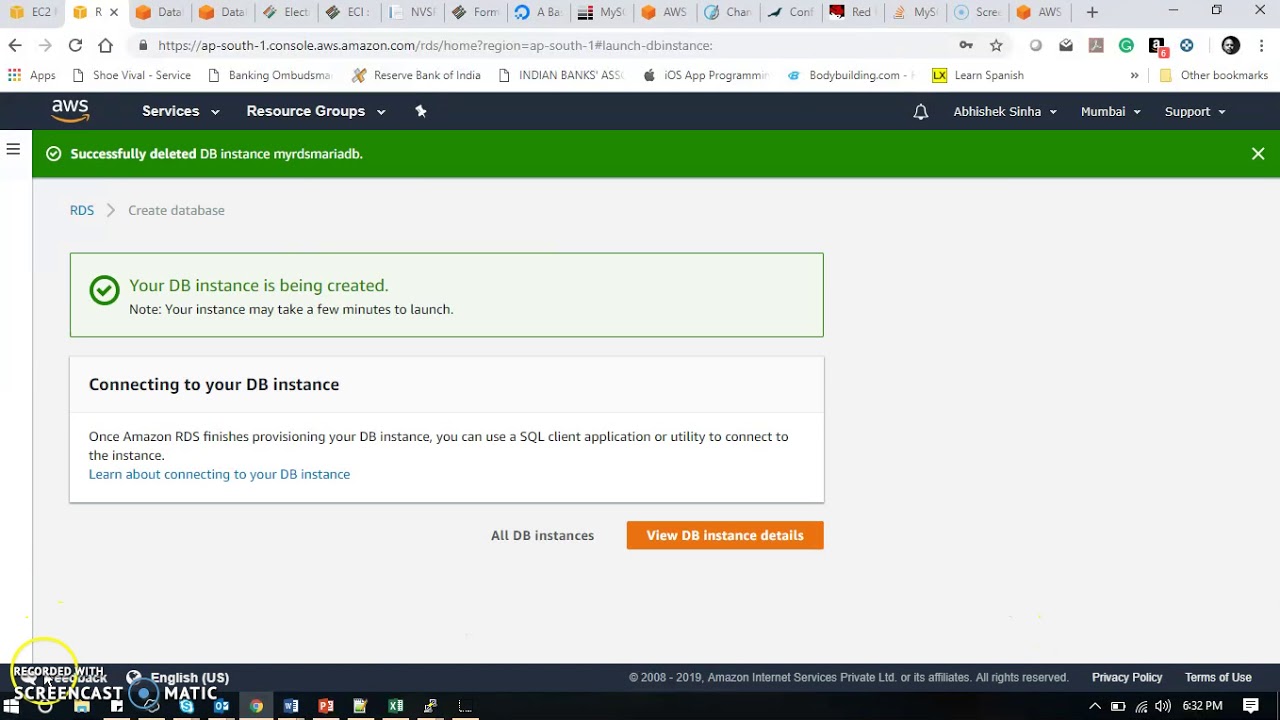Screenshot of an Amazon Web Services (AWS) Management Console

The image captures a section of the AWS Management Console on what appears to be a user account belonging to Abhishek Sinha. 

- **Top Navigation Bar:** 
  - **Left Side:** The AWS logo with the Amazon arrow beneath it.
  - **Center Area:** Several dropdown menus are present: "Services," "Resource Groups," and "Notification Bell," indicating a list of alerts.
  - **Right Side:** User-specific elements including the username "Abhishek Sinha" with a dropdown arrow, "Mumbai" as the selected region with a dropdown arrow, and a "Support" dropdown menu.

- **Notification Section:** 
  - A green notification message displaying "Successfully deleted DB instance," indicated by a white checkmark inside a green circle. To the right of this notification is a closeout cross.

- **RDS Section:**
  - A header labeled "RDS" next to four outward-facing arrows, alongside a button labeled "Create database."
  
- **Progress Notification:**
  - A light green, bordered section with a checkmark stating, "Your DB instance is being created. Note: Your instance may take a few minutes to launch."

- **Connection Instructions:**
  - Below the progress notification, there is a white box with a faint gray border containing the message: "Connecting to your DB instance."
  - Within the box, it details: "Once Amazon RDS finishes provisioning your DB instance, you can use a SQL client application or utility to connect to the instance."
  - A link is provided to learn more about connecting to the DB instance.

- **Action Buttons:**
  - At the bottom of the section, there are two buttons: "All DB instances" and, to the right, an orange button labeled "View DB instance details."

The screenshot comprehensively illustrates the user interface elements related to managing a database instance within AWS, capturing both the navigational structure and pertinent notifications for database management activities.